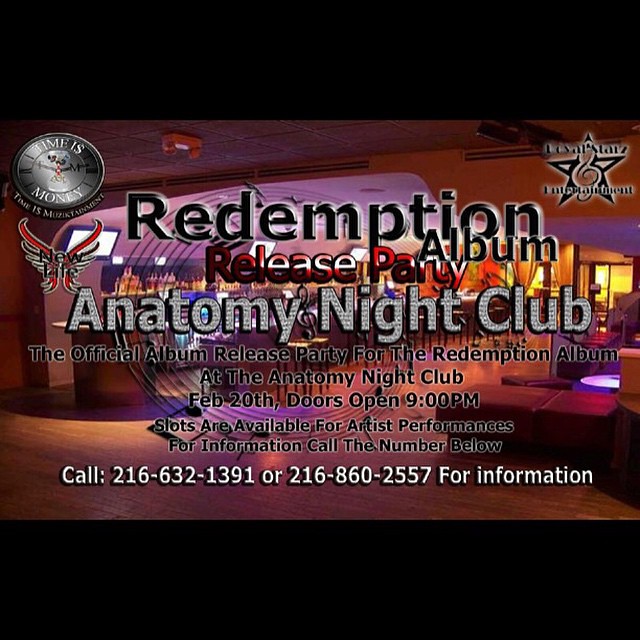The advertisement features a vibrant and detailed nightclub announcement framed by black borders at the top and bottom. The central focus of the image, which occupies about 60% to 70% of the space, is a slightly obscured bar scene illuminated in a mix of purple, orange, and pink hues, capturing the lively ambiance of the club. Prominently featured in this background is a liquor cabinet in front of a mirror, seating for patrons, and a glass door on the right side opening up to a scenic sunset or sunrise view.

Overlaid on this bar scene, in the upper left-hand corner, is an emblem with the text "Time is Money," accompanied by a silver coin logo. On the right side, a black star symbol adds to the festive details. The main event details are highlighted in various fonts and colors: "Redemption Release Party Album" in bold characters on the right, while the event title "Anatomy Nightclub" occupies the center in blocky font. Below, additional event information is provided in a smaller black font: "The official album release party for the Redemption album at the Anatomy Nightclub, February 20th, doors open at 9 p.m. Slots are available for artist performances. For information, call the number below." The contact numbers, presented in white font across the dance floor area, are 216-632-1391 and 216-860-2557.

Overall, the imagery and text combine to create a vivid and informative advertisement for the "Redemption Album Release Party" at Anatomy Nightclub, emphasizing its vibrant club atmosphere and providing essential details for potential attendees.